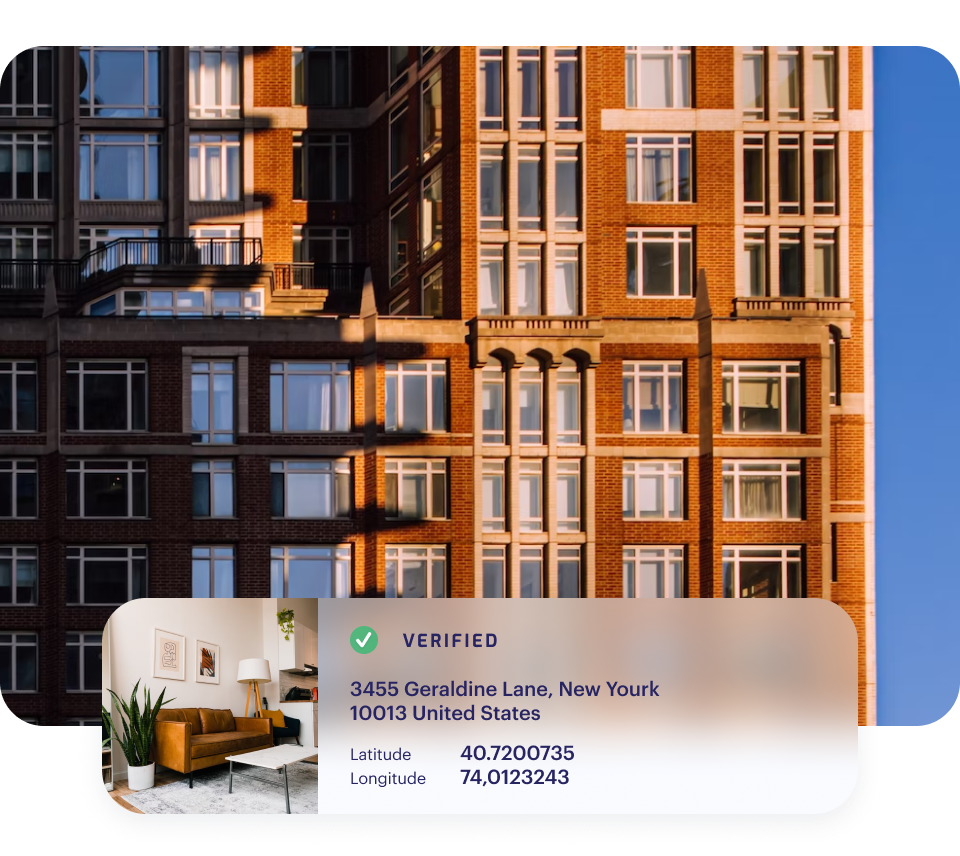The photograph features a prominent building distinguished by its extensive red brick façade and numerous windows framed in white. The building is bathed in sunlight on its right side, while the left side is cast in shadow. Below the main image, there is a semi-transparent white strip resembling frosted glass, which contains important information: "Verify, 3455 Geraldine Lane, New York, 10013, United States, latitude 40.7200735, longitude -74.0123243."

To the left of the information strip, a cozy living room setup is visible. The living room includes a couch, a coffee table, a plant, and a lamp, creating a warm and inviting atmosphere. The photograph showcases a diverse color palette featuring shades of blue, red, white, gray, green, brown, black, and yellow, contributing to the overall vividness of the scene.